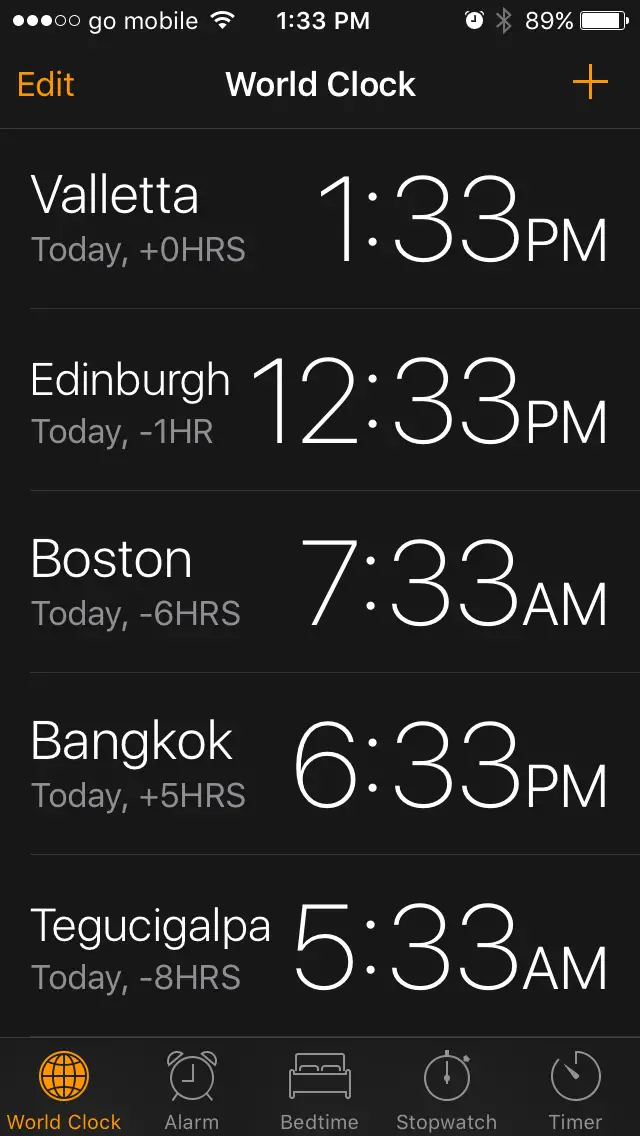The image captures a cell phone screen showing a World Clock application. At the top left, the screen displays mobile network bars labeled "Go Mobile" and Wi-Fi signal strength. The time, "1:33 p.m.," is centered at the top, accompanied by icons for an alarm, Bluetooth, and a battery indicator showing 89% charge. 

Just below this information bar, there's an "Edit" button in orange on the left, and a white-capped text "Roll Clock" next to it. To the right is an orange plus sign ("+"). A gray horizontal line separates this section from the main content.

The main content lists various world cities and their current times. These times are presented with large, bold numbers, the most prominent feature on the screen. Starting with "Valetta," which is spelled out as B-A-L-L-E-T-T-A, it shows it is "Today, plus zero hours," with the time "1:33 p.m." displayed prominently to the right. Subsequent lines show:

- "Edinburgh, Today, negative one hour, 12:33 p.m."
- "Boston, Today, negative six hours, 7:33 a.m."
- "Bangkok, Today, plus five hours, 6:33 p.m."
- "Tegucigalpa, Today, negative eight hours, 5:33 a.m."

At the bottom of the screen, another gray line separates the world clock information from a navigation bar. The navigation options start with "Roll Clock" in orange on the left, followed by gray icons labeled: "Alarm," "Bedtime," "Stopwatch," and "Timer."

The screen features a minimalist color palette comprising white, black, gray, and orange. The time digits are significantly larger than any other text on the screen, with the city names being the second most prominent.